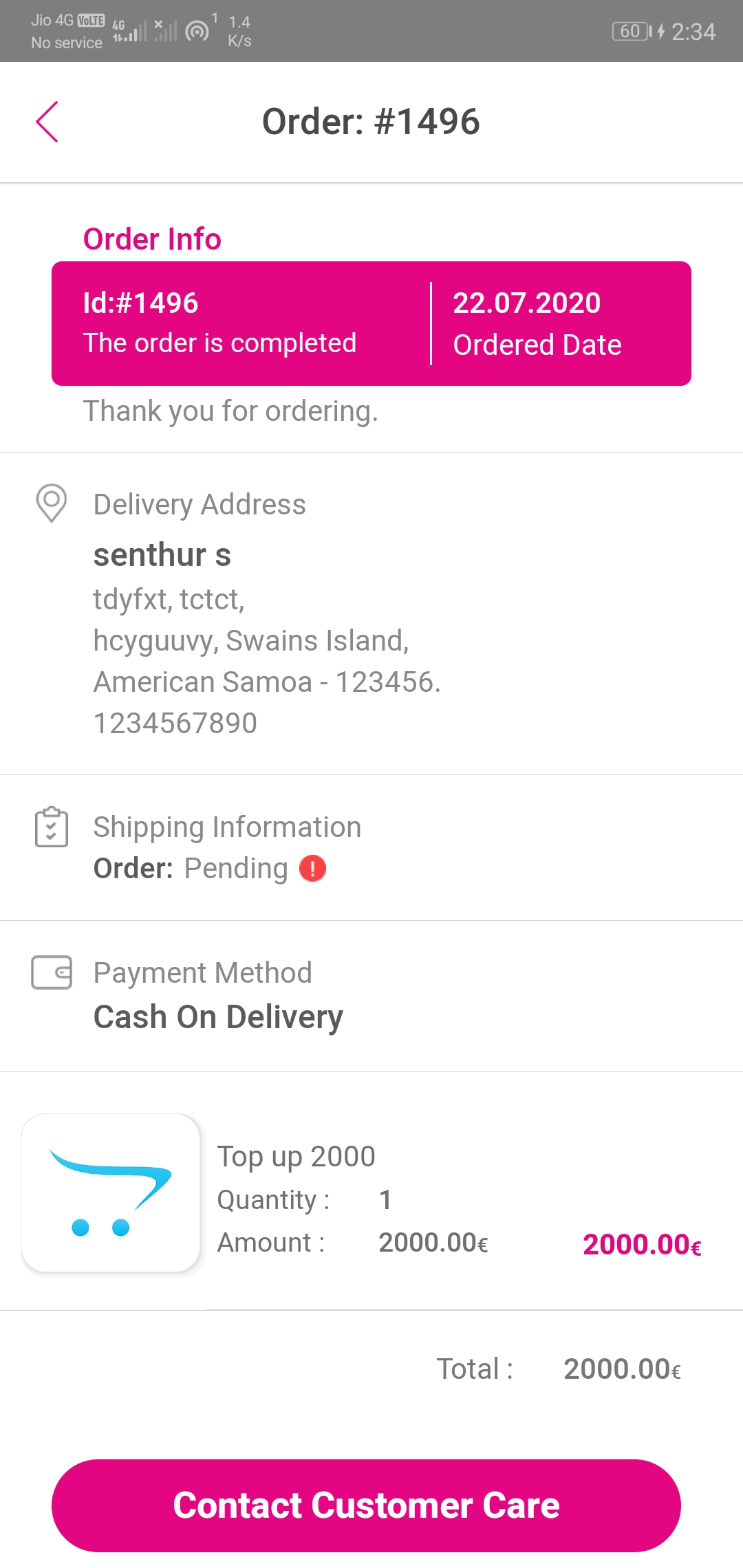This image shows a smartphone screen displaying an app page detailing order number 1496. At the top left corner, a left arrow button indicates that tapping it would return the user to the previous page. The page prominently features a pink box with white text indicating the ID number 1496, and a status message reading "Order Complete." Below this, the order date and delivery information are listed. The delivery address appears fictional and includes random characters before mentioning "Swain's Island, American Samoa." The shipping information section indicates that the order is still pending, while the payment method is noted as "Cash on Delivery." At the bottom of the screen, a pink button labeled "Contact Customer Care" in white text invites users to seek assistance.